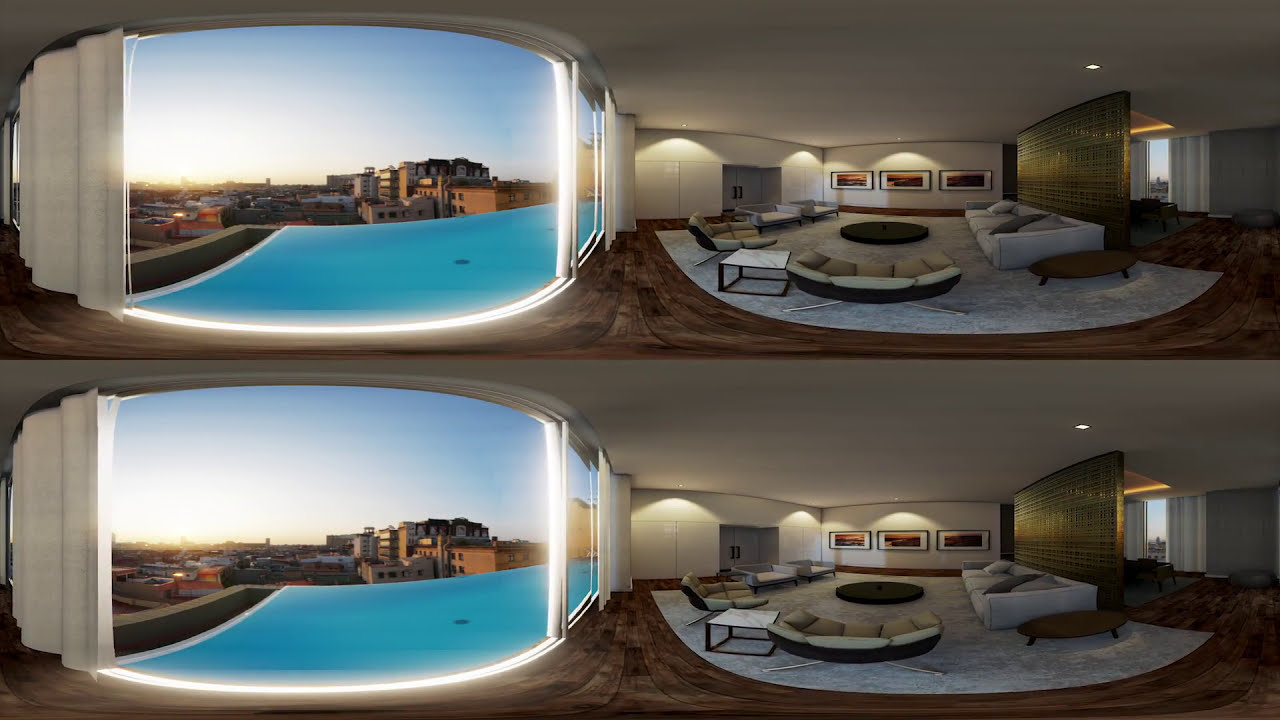The image shows a luxurious living room, duplicated one above the other, each occupying half of the frame. On the left side, a series of large windows reveal an expansive view of a city's skyline, with various buildings ranging from small to large, indicative of an apartment building setting. Outside, rooftops and a pool can be seen. The living room, characterized by its elegant hardwood flooring and a silvery-blue carpet, features spacious furniture arrangements, including two chairs, several love seats, and a large couch positioned against a divider in the middle of the room. This divider separates the living space from another room visible behind it. The right side of the living room displays three paintings on the wall and a pair of outward-opening doors. The ambiance is bright, with well-placed lighting reflecting off clean white curtains drawn to the side.